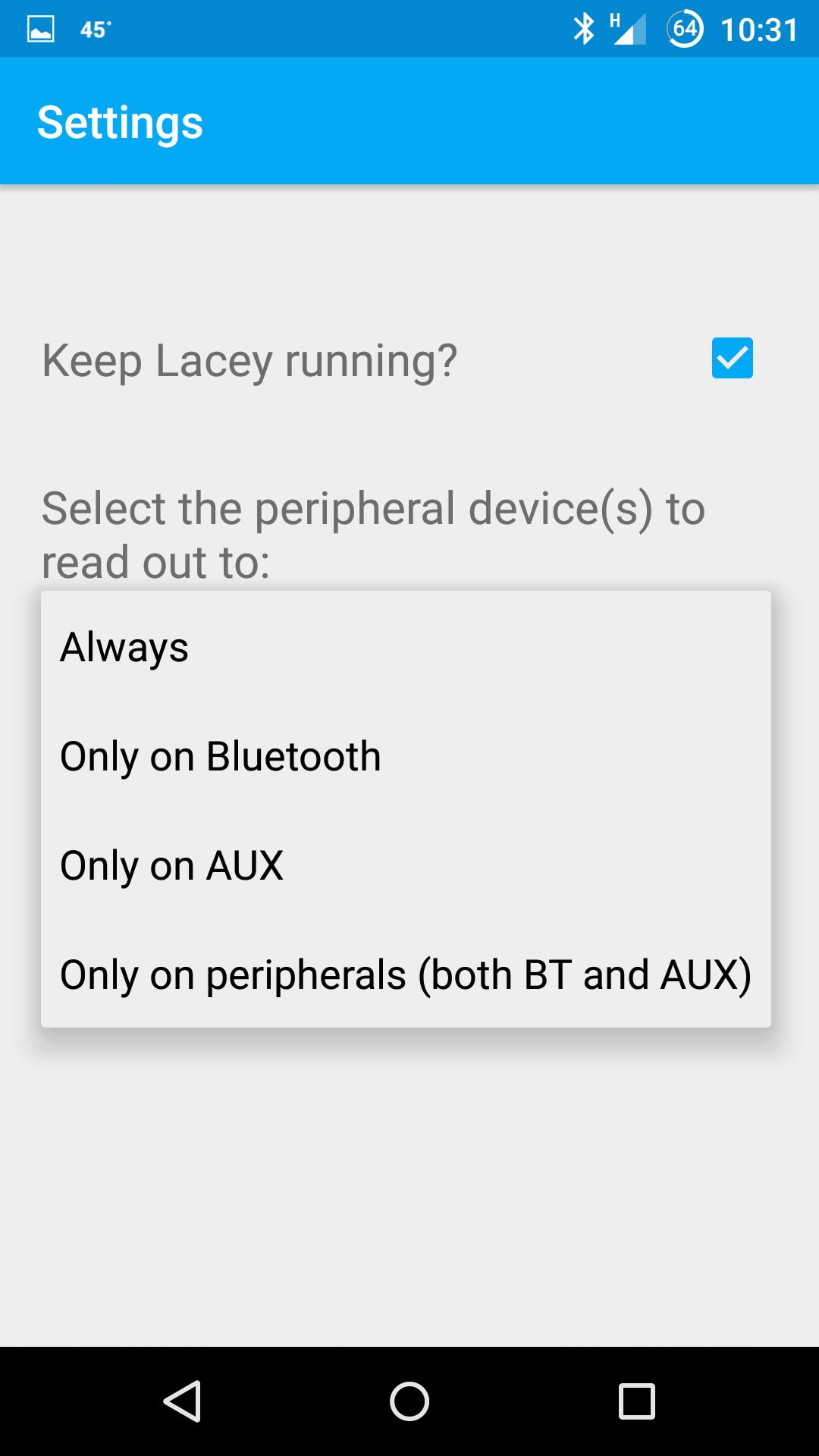Screenshot of a Smartphone Settings Menu

The screenshot captures a smartphone's settings interface, showcasing various details. At the top, the status bar indicates the current temperature of 45 degrees, the time as 10:31, and the battery level at 64%. The status bar features a gradient color design, transitioning from a slight blue to a lighter Carolina blue.

The main settings screen is predominantly gray with the word "Settings" displayed in white text. Just below, a section titled "Keep Lacy Running" shows a checkbox that has been positively checked, marked with a blue checkmark.

Beneath this, there is an option to "Select the Peripheral Devices" with a dropdown menu that appears to list various options. These options include different modes for running "Lacy" through "Always," "Only on Bluetooth," "Only on Auxiliary," or "Both BT (Bluetooth) and Auxiliary."

At the bottom of the screen, enclosed in a black border, are traditional navigation symbols including back and power off/close functionalities.

This screenshot suggests that the user is configuring the settings for a particular function, "Lacy," and deciding under which conditions it should be kept running on their device.